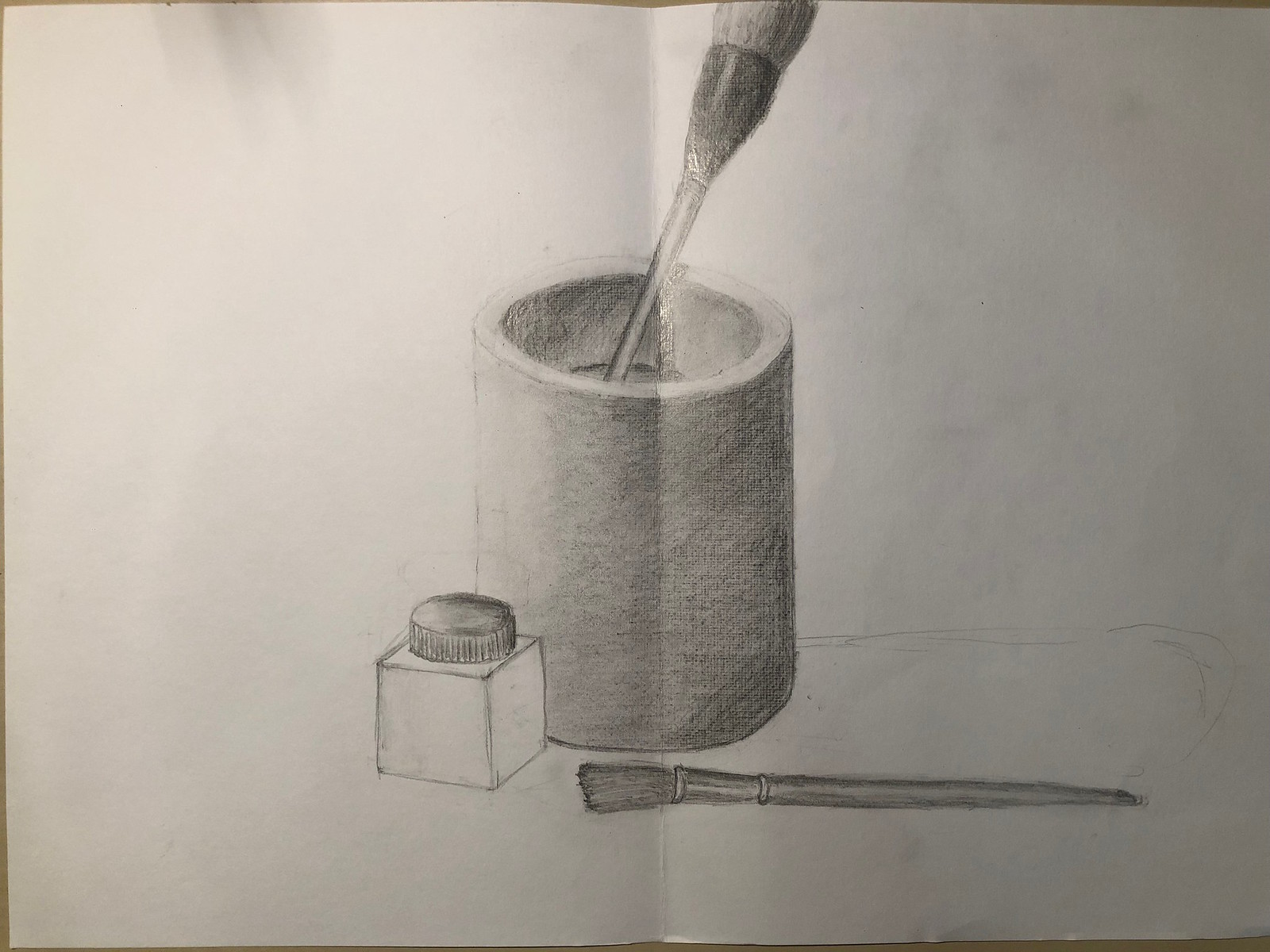This detailed pencil sketch, drawn on a piece of sketch paper folded in half, prominently features a cup depicted in three-dimensional form. The cup holds a single paintbrush standing upright. Positioned in front of the cup lies a smaller paintbrush. Additionally, a small, square-shaped inkwell with a round top is carefully placed against the lower left hand corner of the cup. The composition is further enriched with additional pencil marks above the smaller paintbrush, adding texture and depth to the scene. A visible crease runs vertically down the center of the sketch, marking the fold in the paper.